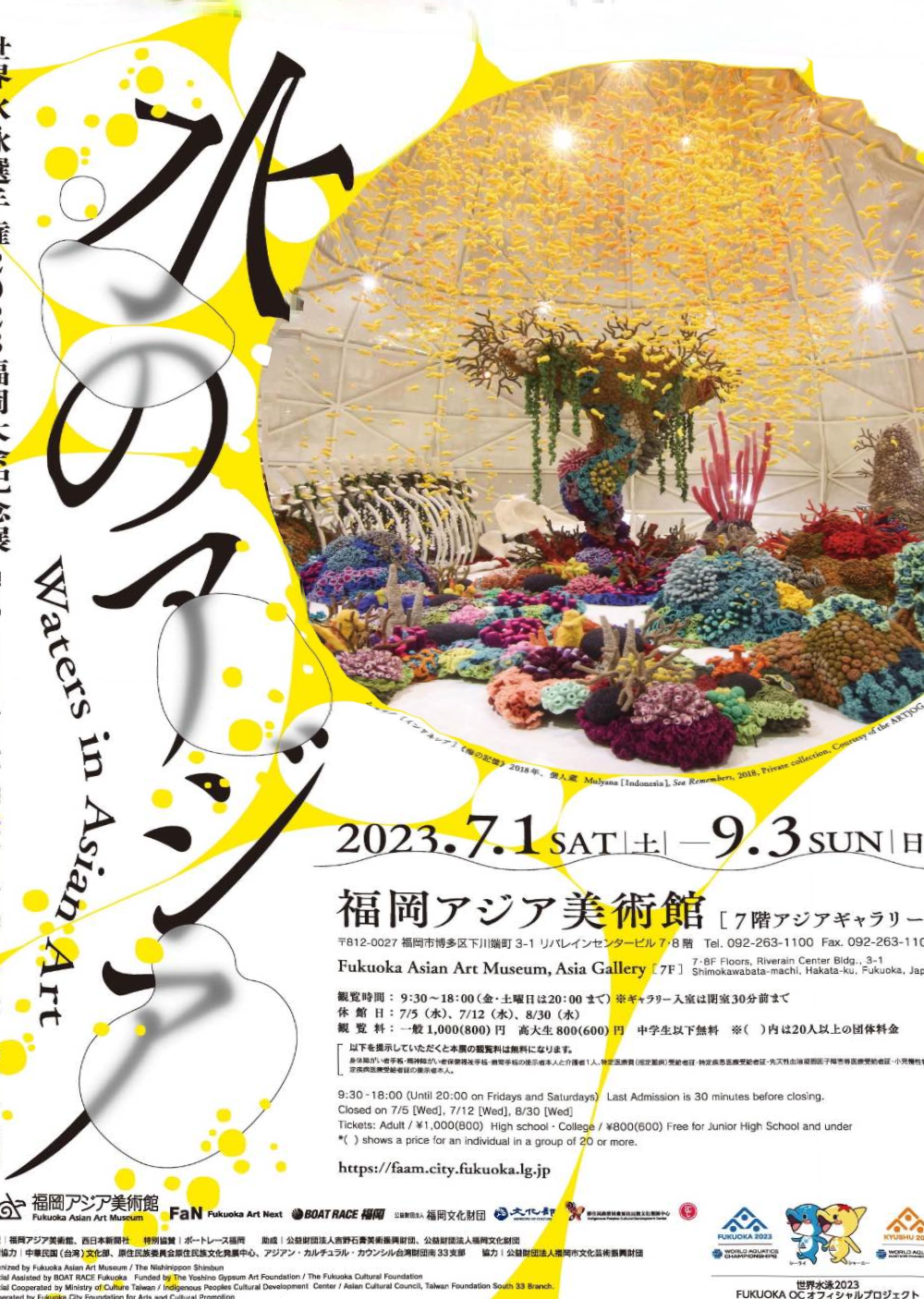This detailed advertisement poster for the Fukuoka Asian Art Museum's Asia Gallery showcases an indoor garden exhibit. Dominating the upper right corner, a circular photograph captures an ethereal indoor space resembling a dome, with a central large, possibly artificial tree surrounded by various bushes, corals, and lush plant life. The white floor is punctuated by the intriguing presence of what looks like a dinosaur rib cage on the far left. Overhead, delicate yellow flowers or perhaps fake butterflies dangle, enhancing the whimsical atmosphere. The poster's design features a predominantly white background adorned with splashes of yellow and semi-transparent bubbles floating upwards. The text, predominantly in Japanese, includes key English details such as the event dates, "2023.7.1 Saturday through 9.3 Sunday," and the venue, "Fukuoka Asian Art Museum Asia Gallery." Logos and additional information are placed neatly at the bottom right, underscoring the poster’s promotional purpose for this Asian art-themed exhibit.